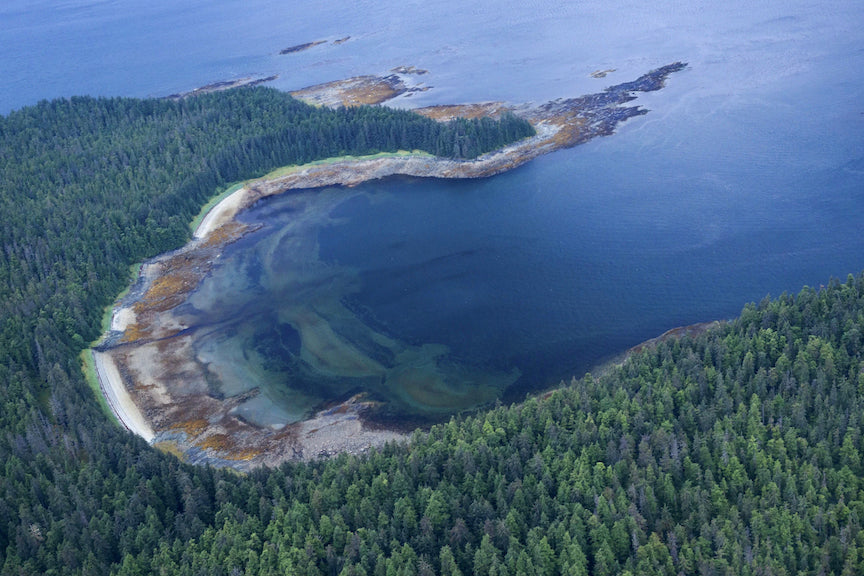This striking aerial photograph, likely captured by a drone or helicopter, showcases a dramatic coastal landscape dominated by a vigorous inlet resembling a horseshoe or the letter "C." The focal point of the image is a natural bay, carved out elegantly by the relentless sea, forming a remarkable peninsula that juts into the water and then curves back. The water itself presents a captivating gradient, starting from deep, pitch-black blue in the deeper sections to lighter greenish hues as it becomes shallower near the shore. 

The shore is characterized by a mix of brownish sandy beaches interspersed with white areas, possibly rocky outcrops or mossy regions. A road traces the circumference of the inlet, hinting at human presence amid the natural beauty. The entire landscape is enveloped in a dense, lush forest, predominantly composed of tall evergreen pines, which add a rich, green texture to the scene. This verdant forest blankets the landmass that stretches across the bottom and right of the picture, emphasizing the area's forested expanse. The distinct geological features of the formation suggest a volcanic origin, adding to the mystique of this picturesque coastal enclave.